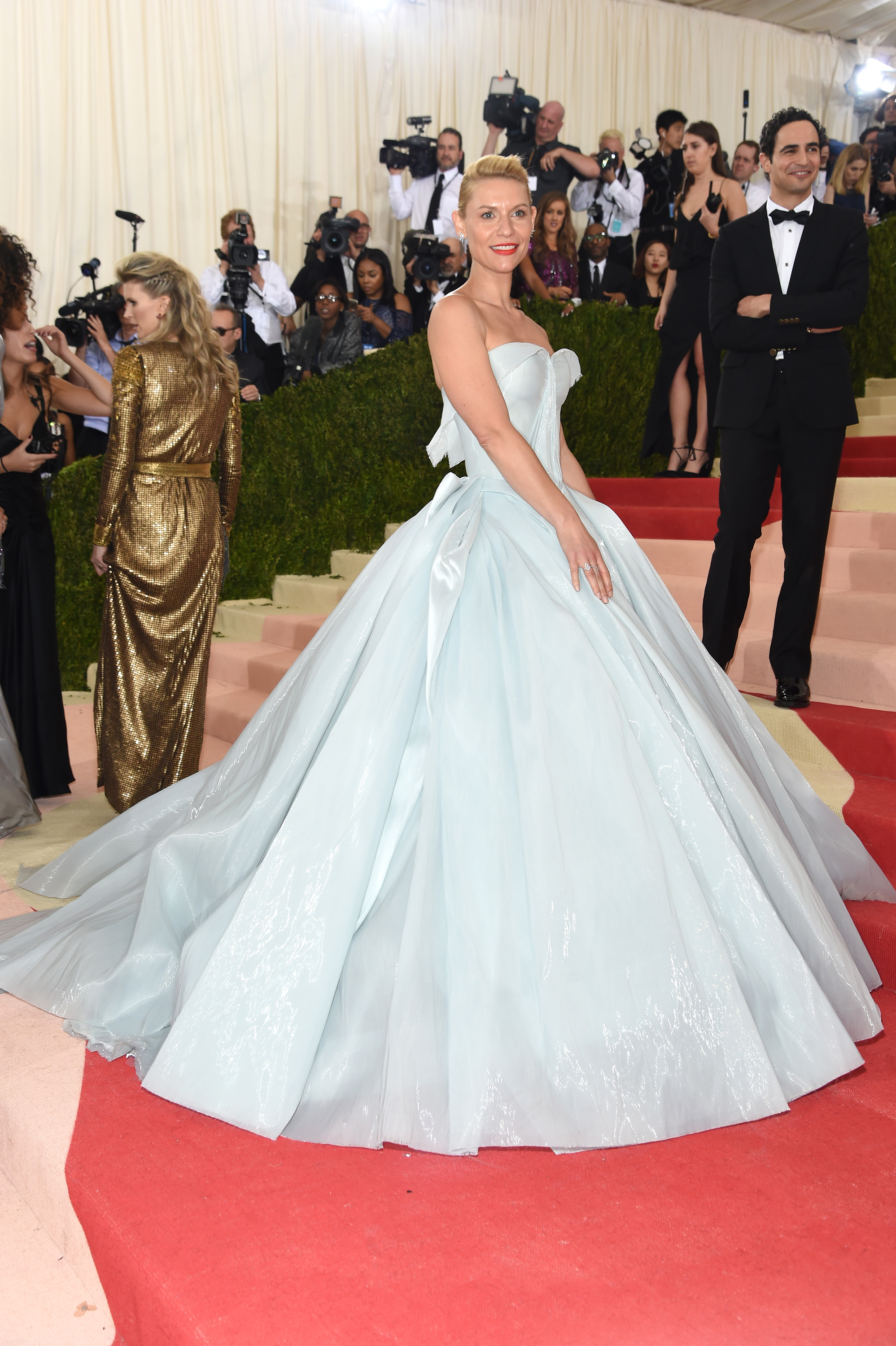In this photograph, a woman stands elegantly on a red carpet, likely at an awards show or gala event. She gazes directly at the camera with a confident smile. Her body is slightly turned to the right, showcasing her stunning, large white sleeveless dress that flows into an extravagant bell-shaped skirt. Her blonde hair is styled up, and she wears prominent red lipstick with no visible jewelry. 

To her right, a man in a black suit, white shirt, and black bow tie stands on a staircase, his hands folded and a smile on his face. He appears slightly balding. A woman in a gold-colored dress that reaches her ankles is also visible in the background, engaged in conversation with another person. This woman, also blonde, is standing near the staircase covered by cloth.

The backdrop of the scene includes low green bushes and a bustling crowd of paparazzi and press photographers, all eagerly capturing the moment. The sheer number of photographers and the formal attire of the attendees underscore the importance of the red carpet event.